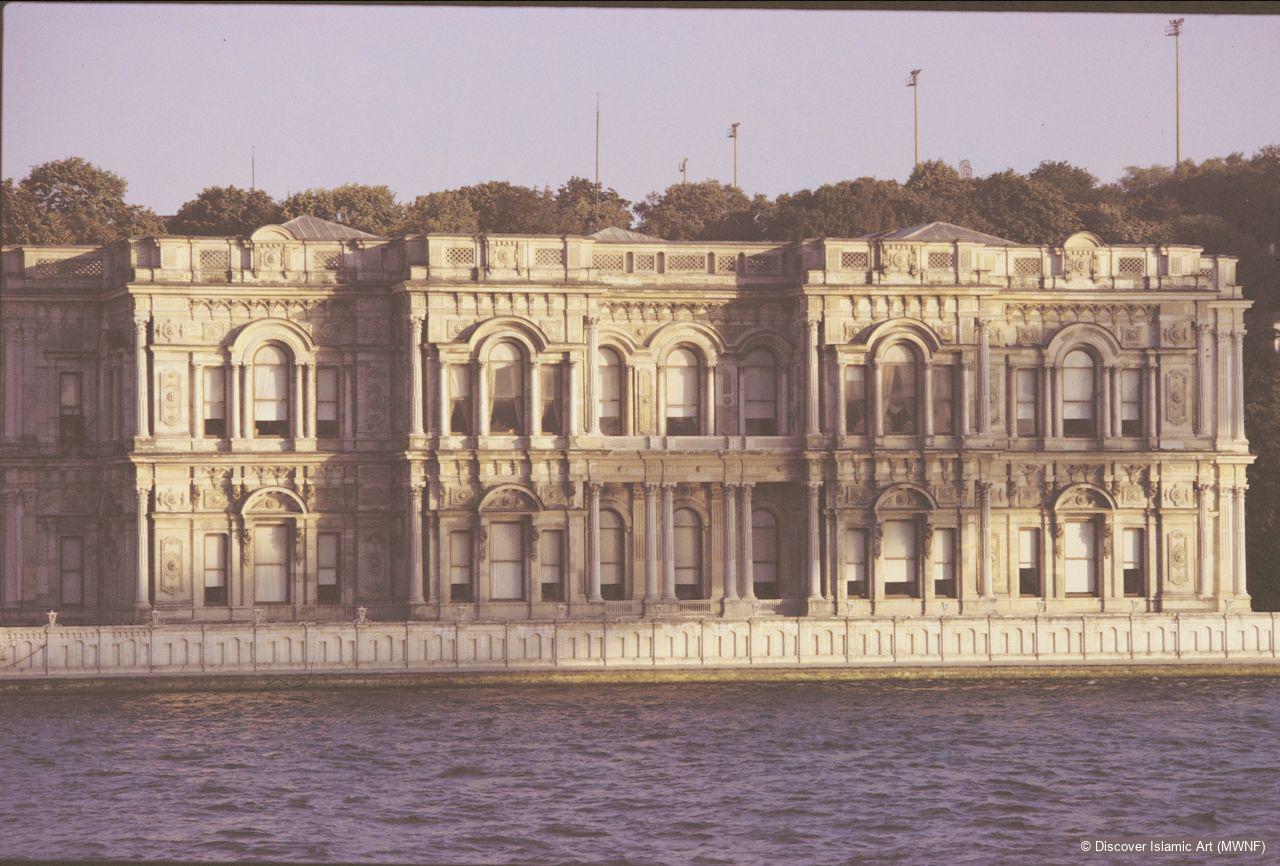The image depicts an old, grand building made of white or beige stone, likely marble, situated on a waterfront. The structure exhibits a classic architectural style reminiscent of Roman or Grecian temples but is identified as Islamic art, as noted by the watermark in the bottom right corner that reads “Discover Islamic Art (MWNF).” The building features numerous arched windows and doorways, arranged in three main sections that are slightly offset from one another, creating a tiered appearance. The facade suggests a two-story height, capped with a pointed turret at the top. The surrounding environment includes a tranquil river or lake in the foreground and mature trees and possibly flagpoles or light posts in the background. The sky has a purple-gray hue, implying either dusk or a brewing storm, and the overall coloring of the photograph has a desaturated, sepia-like tint with an orange-red tinge, adding to the aged and serene atmosphere of the scene.